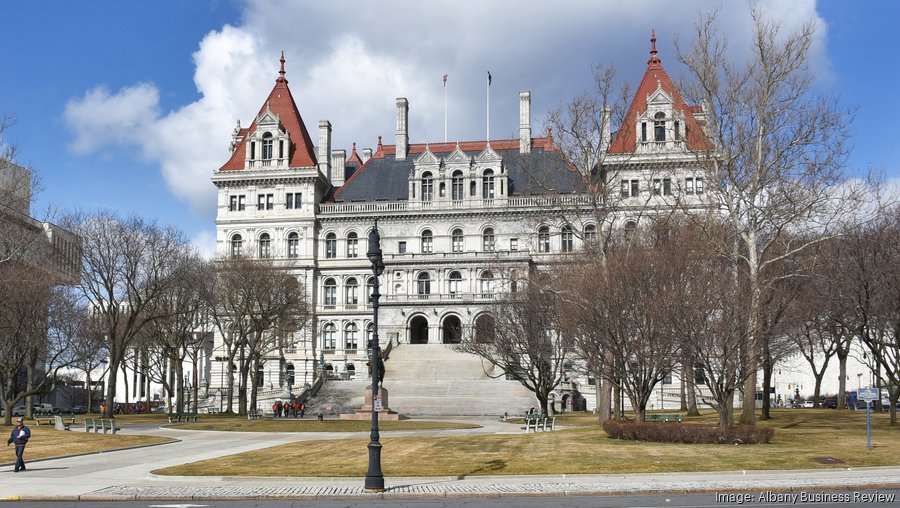The photograph, credited to the Albany Business Review, captures a stately multistory building facing directly towards the viewer. This imposing structure appears to be a restored historical edifice, possibly dating back to the 19th century, and is characterized by its white walls and brown tiled roofs. It features a central horizontal portion with four stories, the fourth story adorned with three arched vertical windows. The building's design includes elaborately carved fake columns, dome-shaped windows with flat bottoms, and prominent red-trimmed roofs with steep slopes and white chimneys on either side.

A broad set of concrete steps leads up to three large, archway entries, emphasizing the building’s grand entrance. The scene takes place in winter, evident from the leafless trees and the brownish-green grass that surrounds the area. A circular driveway encircles a statue—possibly a winged horse—positioned centrally in front of the building, adding a historical significance to the square. The sky, a patchwork of white and dark clouds, forms a dramatic backdrop to the pale building and amplifies its majesty. People can be seen walking around the site, enhancing the scene’s liveliness despite the season’s dormant foliage. Benches and flagpoles add functional and aesthetic touches to the surroundings.